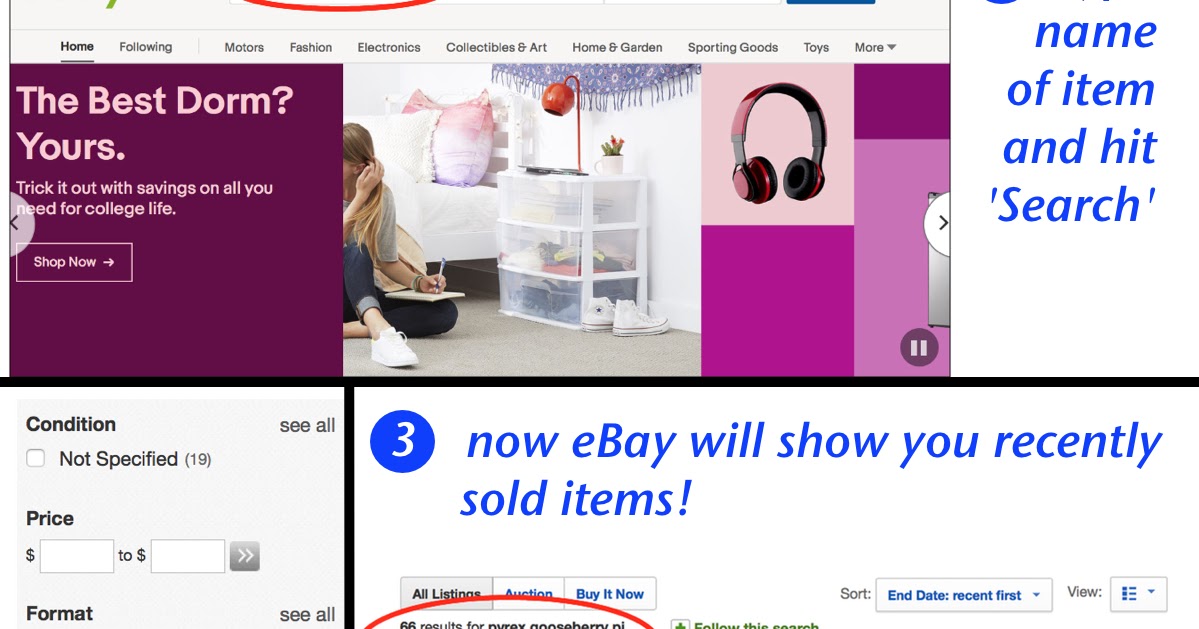Here is a cleaned-up and detailed caption for the given image description:

---

The image depicts a predominantly purple-themed website layout with white accents. At the top of the page, there is a navigation bar with labels for different categories including "Home," "Following," "Motors," "Fashion," "Electronics," "Collectibles and Art," "Home and Garden," "Sporting Goods," "Toys," and "More." A promotional banner appears below, reading "Trick it up with savings on all you need for college life."

On the left side, there are purple squares interspersed in the design, drawing attention to key areas. One of these squares is centrally placed. In the middle of the page, a woman with long hair is sitting on a chair, writing in a notebook. Next to her is an organizing cabinet with a lamp perched on top of it. Various elements, including a pink pillow and a set of headphones, add character to her workspace.

Further down the page, there is a red, white, and blue square featuring the name of an item and a search bar. At the bottom left, there is a section labeled "conditional specified CEO price" with directional arrows. A large circle with the number three inside it is prominently displayed to the right.

Additionally, the page displays options to view sold items with a bracelet shown as an example. Below this, there are tabs for "All Listings," "Auction," "Buy It Now," and a sorting option labeled "Date recent first." Near the bottom, the text "Results for..." is visible, suggesting a listing inquiry, followed by miscellaneous text and images that indicate various types of listings and website elements.

---

This revised caption provides a detailed and structured description of the website layout and its key features.